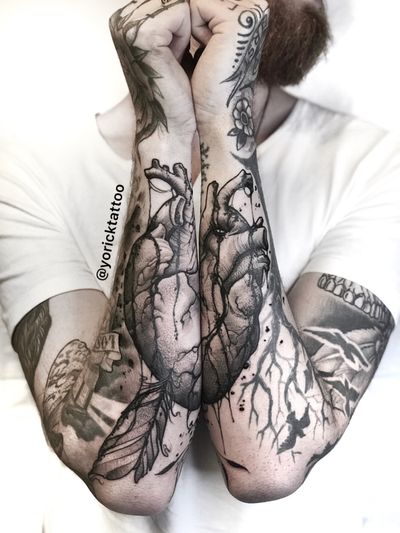In this black and white photograph, a person with long hair, gender unclear, faces the camera wearing a scoop neck white t-shirt. Their hands are held together in front of their face, obscuring it, with their fists balled up and pinky fingers pointing towards the camera. Their elbows are pressed together, causing their arms to merge into a unified display to showcase an intricate tattoo. The tattoo spans both arms, with each half residing on each arm. When the arms are together, the tattoo forms a detailed image of an anatomically correct heart.

This heart-shaped tattoo is detailed with aortas or valves extending from the top of the heart onto the upper portions of the arms. The lower parts of the tattoo, near the elbows, depict an elaborate network of veins fanning out across the arms. Additional elements, such as birds, are visible on the upper right arm. The tattoo includes a copyright text along the left forearm which reads "Yorick Tattoo," suggesting the artist's identity. Despite the ghoulish and striking nature of the tattoo, its craftsmanship is notable, blending realism with artistic depth, likely intended for those seeking detailed and thematic body art.